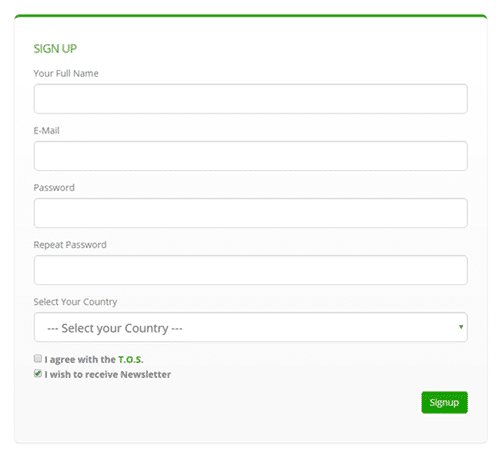This image shows a screenshot of a sign-up form on a mobile device. The form features a thin, gently curved green header at the top of the screen. Below the header, there is a clean white background with labeled input fields outlined in thin gray lines and featuring curved corners. 

The labels for the input fields, written in light gray font, include:
1. Your Full Name
2. Email
3. Password
4. Repeat Password
5. Select Your Country (with "Select your country..." in the placeholder text and a dropdown arrow on the right side)

Beneath the input fields are two checkboxes with accompanying text. The first checkbox, labeled "I agree to the TOS" (with "TOS" in green), is unchecked. The second checkbox, labeled "I wish to receive Newsletters" (with "Newsletters" capitalized), is marked with a green check.

At the lower right-hand side of the image, there's a bright green rectangular sign-up button, matching the color of the header line and TOS text. The button has rounded corners and features "Sign Up" in white or possibly light gray text.

The overall design is clean and modern, emphasizing ease of use and clarity.